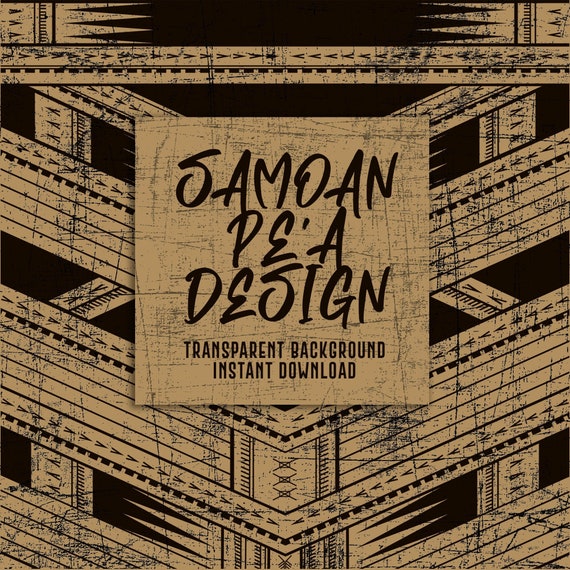The image is a detailed graphic banner with a tan and black color palette featuring a central square sign. The sign prominently displays the text "SAMOAN PE'A DESIGN" in large, black, capital letters that resemble a sharpie handwritten font. Below this main text, in smaller black letters, are the words "Transparent Background Instant Download." Overlaying the entire design is a weathered, scratched filter that gives the image an aged appearance. The background showcases a symmetrical pattern of geometric shapes and lines, forming a series of chevrons that angle downward towards the center and then back up. This pattern is set against a beige and black backdrop with the design extending into brown structures in the background, intersected by black lines that continue the theme of the graphic. The image is well-lit with natural lighting, highlighting the clear and detailed Samoan-inspired design.